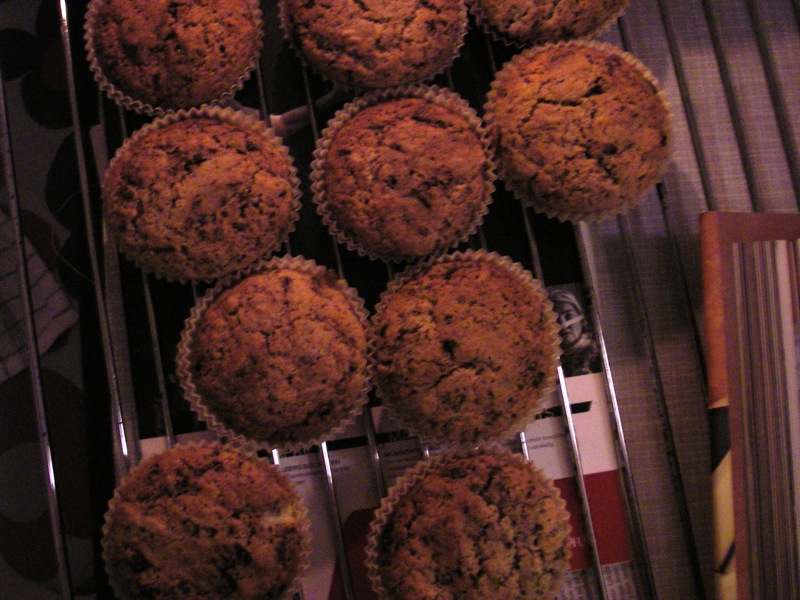This is a top-view photograph of ten muffins cooling on a metal rack. Despite the poor lighting and slight blur, the muffins in their paper cups, some of which appear doubled, can be distinctly seen arranged in rows of varying numbers. They have a brownish hue with visible cracks, suggesting they could be banana or vanilla chocolate chip muffins. Beneath the cooling rack, a dark table is just perceptible, without visible details due to the light quality. On the left, part of a tea towel is peeking out under the metal rack. Behind the muffins, there is a piece of paper or cardboard with red, white, and black details, including a black and white photograph of a woman's face. To the right, next to the rack, there appears to be a wooden object and a possible tablecloth.